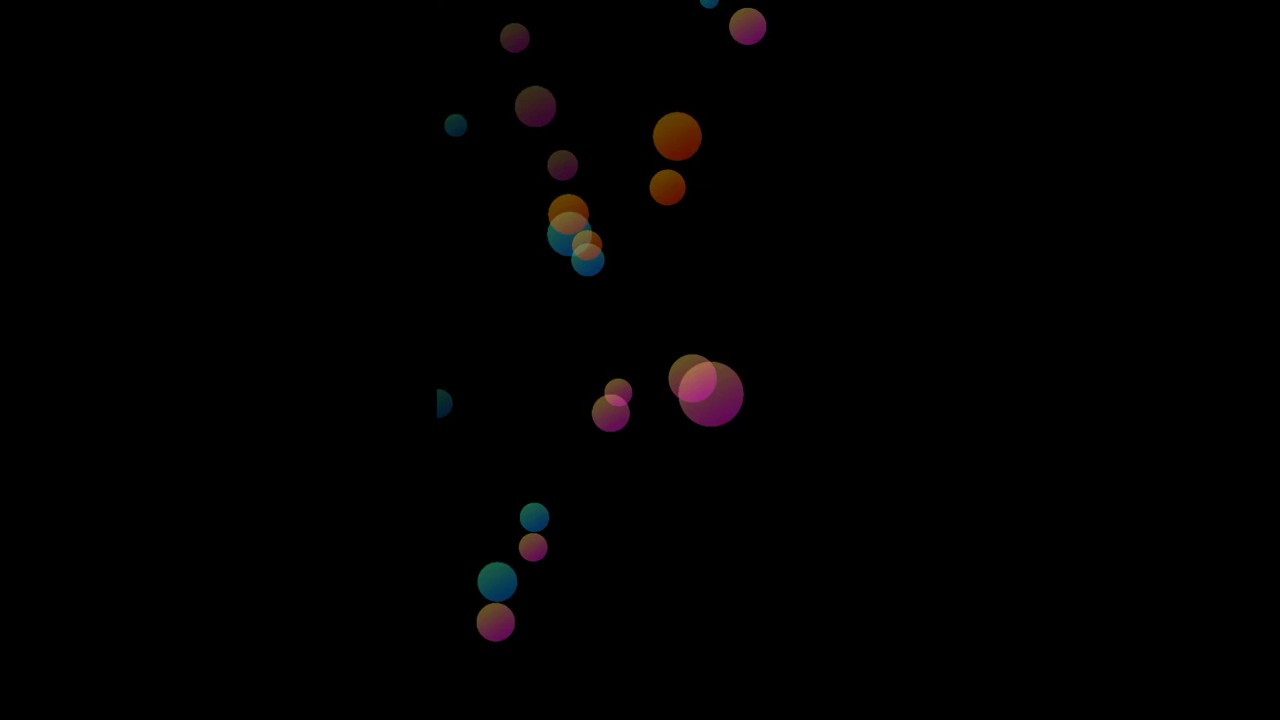In the center of a predominantly black, rectangular image, a collection of multicolored dots—ranging in size and appearing somewhat random and floating—captures attention. These dots, which evoke the appearance of illuminated bubbles, are clustered mainly from the top middle of the image down to the bottom middle, with some extending slightly to both sides. The topmost dots are small and pinkish, giving way to a sequence below: a small blue dot beside a pink and an orange dot, followed by a slightly larger orange dot to the right. Further down, there's a small orange dot adjacent to a purplish one, with a mix of small blue and orange dots interspersed along the column. Notably, there's a unique semicircular blue dot towards the lower center. Some dots blend and overlap, creating a subtle glow where their colors merge. The rest of the image remains a solid black, enhancing the floating, ethereal quality of the luminous dots.